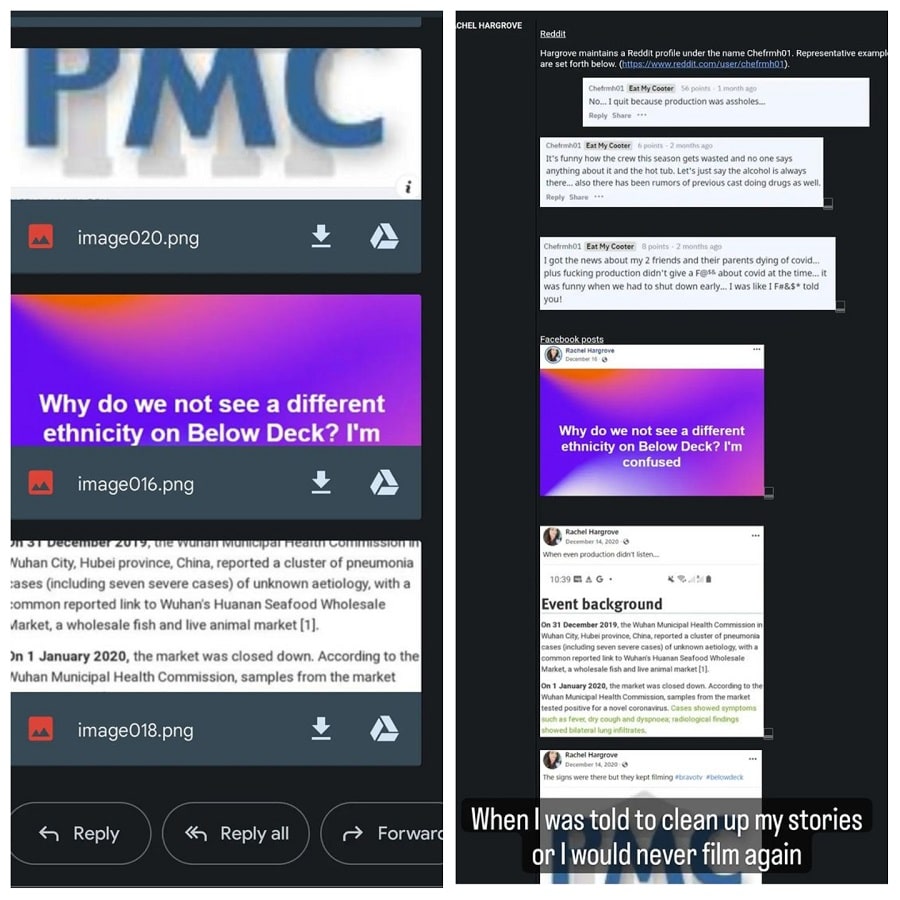The image is a detailed screenshot featuring two vertical sections side-by-side. The left section has a black background displaying several attached images from a Gmail email. At the top, the first image is labeled "image 0.png" and showcases a white background with "PMC" written in blue. Below it, an image with a purple background and a streak of orange at the top poses a question, "Why do we not see a different ethnicity on Below Deck? I'm". The final attachment, "image 018.png," contains an article excerpt discussing COVID-19: "The Wuhan Municipal Health Commission in Wuhan City, Hubei Province, China, reported a cluster of pneumonia cases, including seven severe cases of unknown etiology, with a common reported link to Wuhan's Yunnan Seafood Wholesale Market's Wholesale Fish and Live Animal Market."

The right section of the screenshot appears to reveal part of a Reddit post. The post mentions a user named Hargrove who operates under the Reddit profile "CHEFRMH01." It includes representative quotes such as, "No, I quit because production is assholes," and comments on the crew's behavior: "It's funny, the crew this season gets wasted and no one says anything about it in the hot tub. Let us say the alcohol is always there. Also, there have been rumors of previous cast doing drugs as well."